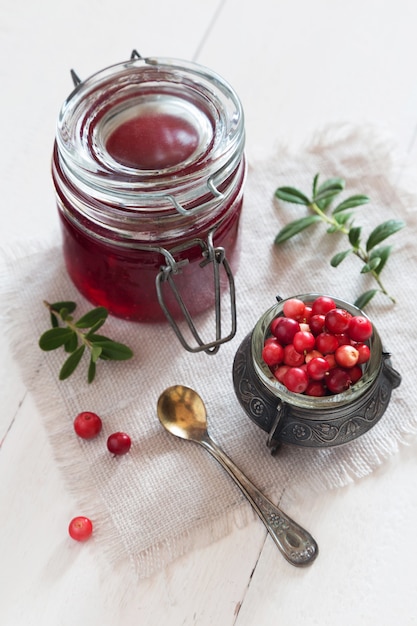This professional daytime photograph captures a meticulously arranged setting featuring vibrant cranberries and a jar of cranberry preserves. The composition, bathed in natural sunlight, centers on an open glass jar filled with a red jelly-like substance, with a few cranberries spilling out onto a white-stained wooden surface. A small pewter or ceramic cup brimming with fresh, glistening cranberries sits near the jar, accompanied by sprigs of greenery. A silver spoon lies next to the cup, and the entire arrangement rests atop a light-colored cloth on the wooden surface. Additional cranberries are scattered around, adding to the rich, inviting display. The color palette includes striking reds, greens, silvers, grays, blacks, whites, and tan, contributing to the image's bright and aesthetically pleasing appearance, suggesting it is a carefully styled, top-down shot with a hint of a front view.